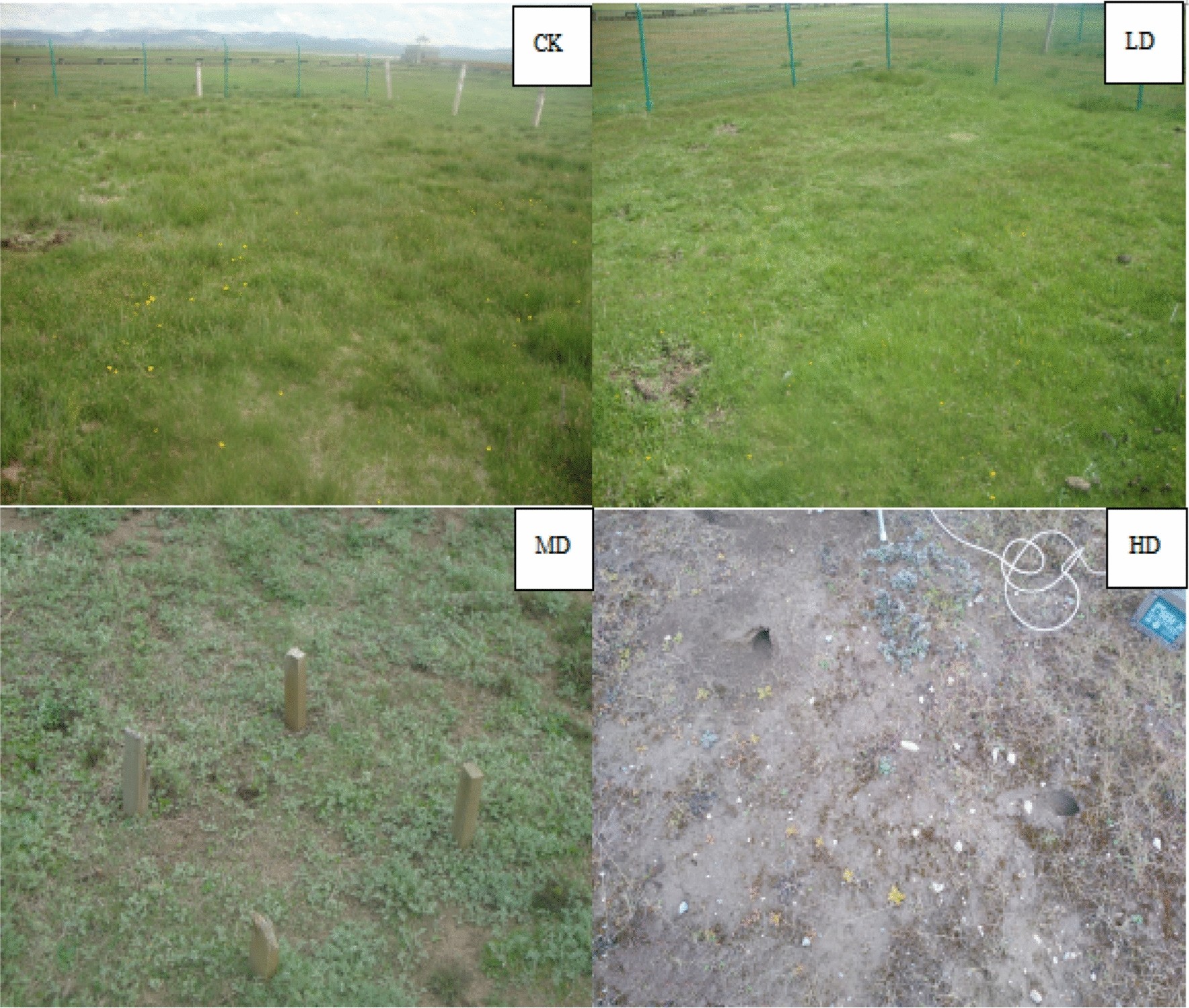The square image is divided into four smaller boxes arranged in a 2x2 grid, each with a distinct outdoor scene and labeled in the upper right-hand corner with black text in a white square. The top left picture, labeled "CK," depicts a field of lush green grass dotted with dandelions, set against a backdrop of purple mountains and a white sky. There is a green fence encircling the area. The top right image, labeled "LD," appears to capture the same grassy area and green fence but from a slightly different angle, maintaining the vibrant greenery. The bottom left picture is labeled "MD" and focuses on the ground, showcasing an up-close view of wooden posts amid soil, with some ground cover plants visible. Lastly, the bottom right image, labeled "HD," presents an almost barren plot of soil with minimal grass, featuring a white cord and a partially visible small blue and gray object. The progression from lush grass to bare soil in the images suggests a study or comparison of different grass growth stages. The predominant colors across the images are black, white, gray, brown, green, and yellow.